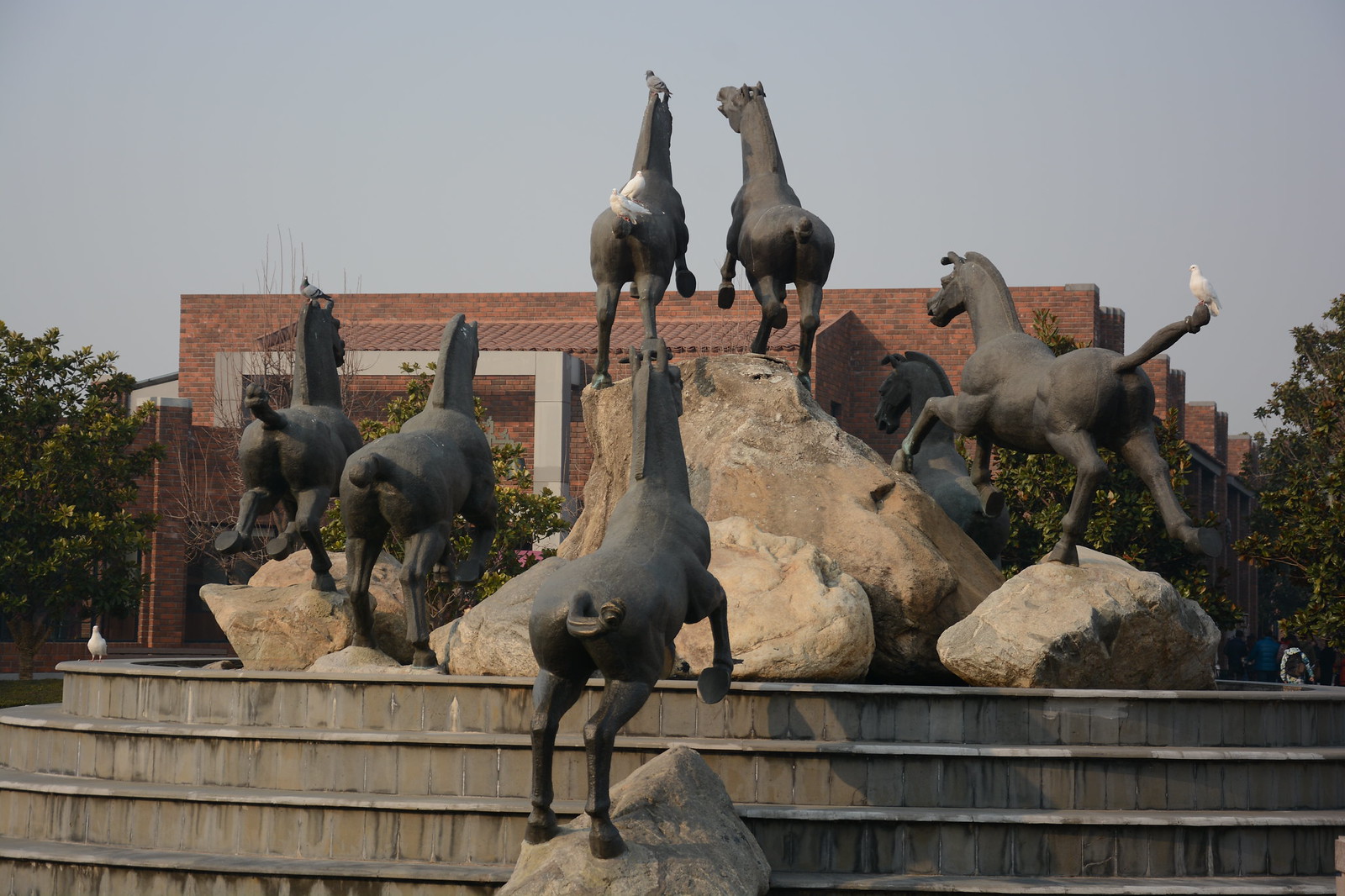In this image, we see a monumental art piece that appears to be a grand fountain, prominently featuring statues of horses in dynamic poses of galloping and climbing. The scene is set on a large structure composed of light brown boulders, forming the base, with the dark gray, almost black horse statues placed atop these stones. Some of the horses have white and gray doves or pigeons perched on them, adding to the intricate detailing.

This impressive fountain is situated in what looks to be a central location of a building complex, possibly within a historical downtown center or a university campus. The entire sculpture rests on a pedestal designed to resemble steps or stairs, indicating a deliberate and artistic elevation. The photo is taken from an angle that emphasizes the back of the horses, which are positioned towards the highest peaks of the stones, giving a sense of upward motion and grandeur.

In the background, a brick building is partially visible, framed by trees with lush green foliage, set against a dusky blue sky devoid of clouds, adding depth and context to the monumental display. The intricate details and the positioning of the elements make this fountain a stunning centerpiece in its environment.